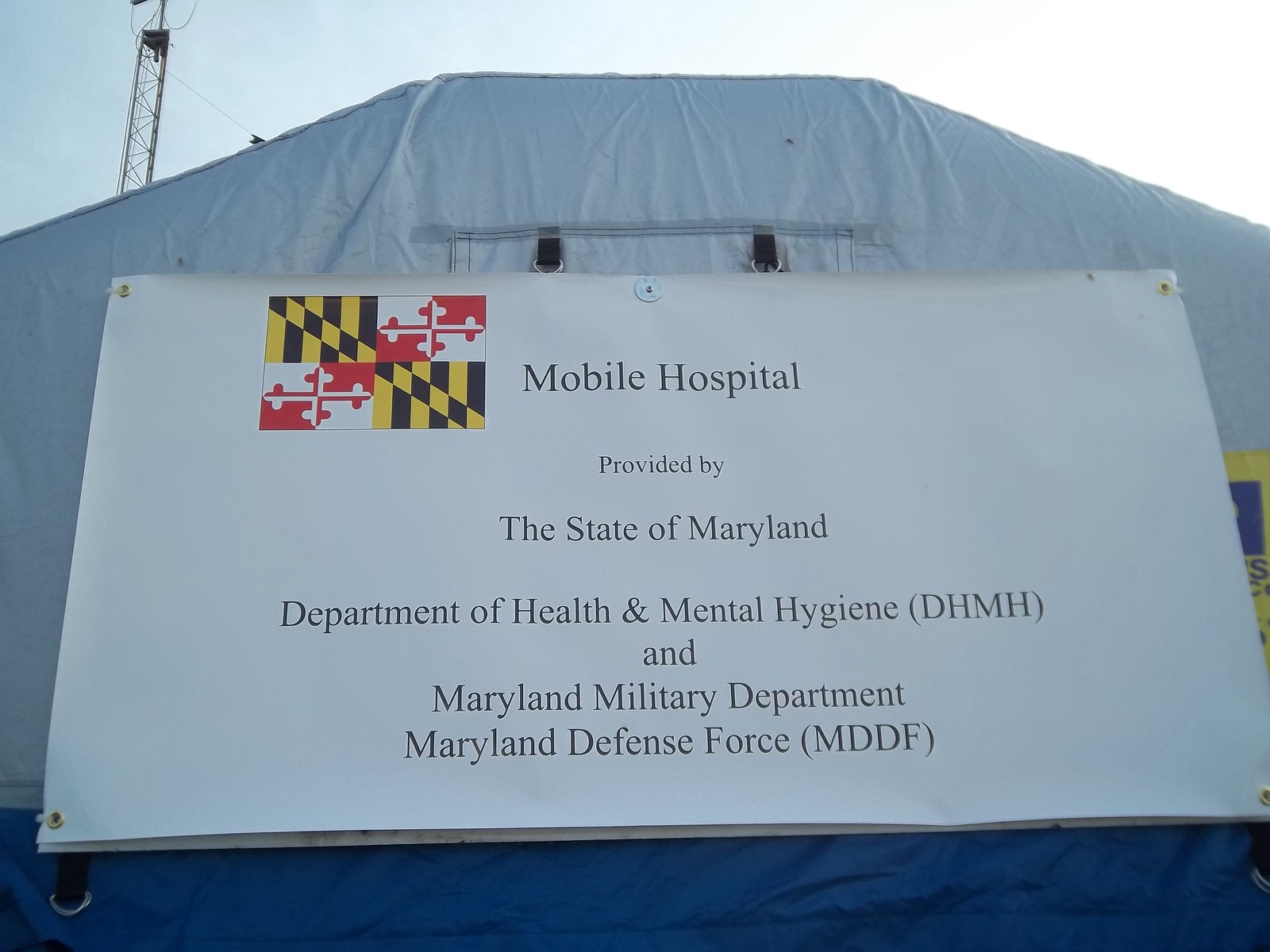This outdoor photograph captures a large tent with a prominent white peaked roof made of thick, heavy canvas and dark blue sides. Suspended on the exterior of the tent is a white sign with a large horizontal rectangle shape. The sign features a logo in the top left corner, composed of a yellow and black checkerboard diagonal line intersected by a red line resembling a medical insignia. To the right of the logo, centered horizontally, the black text reads "Mobile Hospital." Below this inscription, in smaller black text, the sign states "provided by," followed by a larger black text line that reads "The State of Maryland." Continuing below, the text lists:

- "Department of Health and Mental Hygiene (DHMH)"
- "Maryland Military Department"
- "Maryland Defense Force (MDDF)"

The sign is bordered by a gray frame. In the background behind the tent is a clear blue sky, with a tall metal radio tower visible above the left side of the tent's roof. This setup suggests the tent may serve as a temporary medical facility, possibly established for a health emergency like COVID-19.